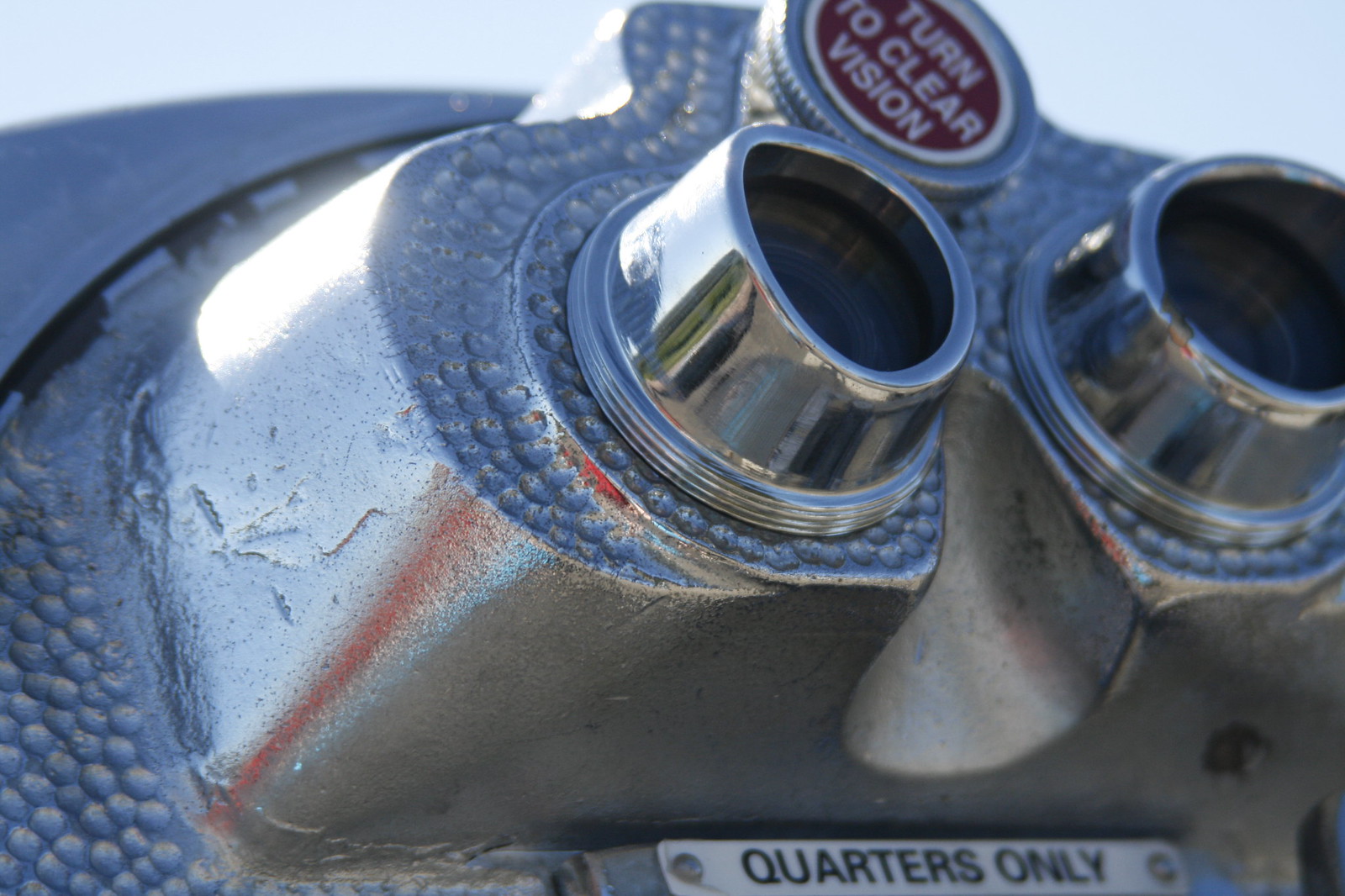This is a detailed close-up photograph of a commercial pay-to-view binocular device, often found at landmarks, zoos, or scenic viewpoints for tourists and visitors to see distant objects. The binoculars are chrome or silver in color with a textured pattern of tiny divots. The image focuses on the eyepieces where users position their eyes. Above the eyepieces, there is a circular red sticker with a white border and white text that reads "Turn to Clear Vision," indicating the focus knob. Below the eyepieces, at the very bottom of the photograph, there is a small sign that reads "Quarters Only," denoting the coin-operated mechanism that allows use of the binoculars. The background of the image is a clear sky, providing contrast to the chrome detail of the viewfinder.